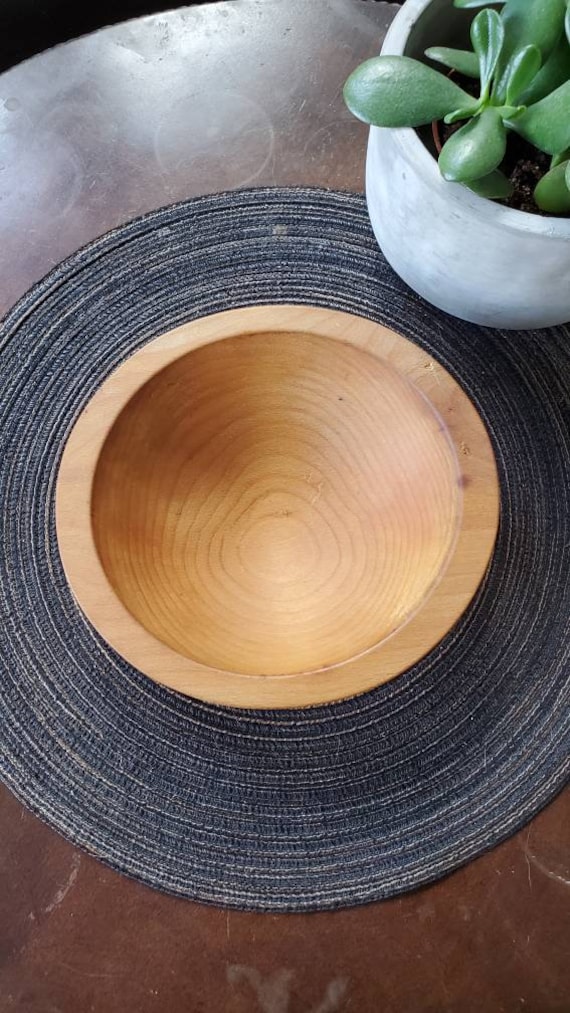This photo features a small, circular table with an old, dingy surface marked by water lines and scratch marks, indicating wear and tear from use. The table is visually divided into sections: the outer edge is a dark brown color, while the middle section consists of fabric-like layers arranged in concentric circles. The innermost section forms a recessed semicircle, slightly lowering the center of the table. 

On the tabletop, a monochromatic woven placemat in black and dark gray tones, interspersed with bits of white and various shades of gray, stands out. Placed atop this mat are two distinct items: a white clay planter holding a few sprigs of a green jade plant occupies the top right corner, and an empty wooden bowl is centrally positioned. The photograph lacks any additional objects, text, or individuals, focusing solely on these central elements on the aged, stained surface of the table.